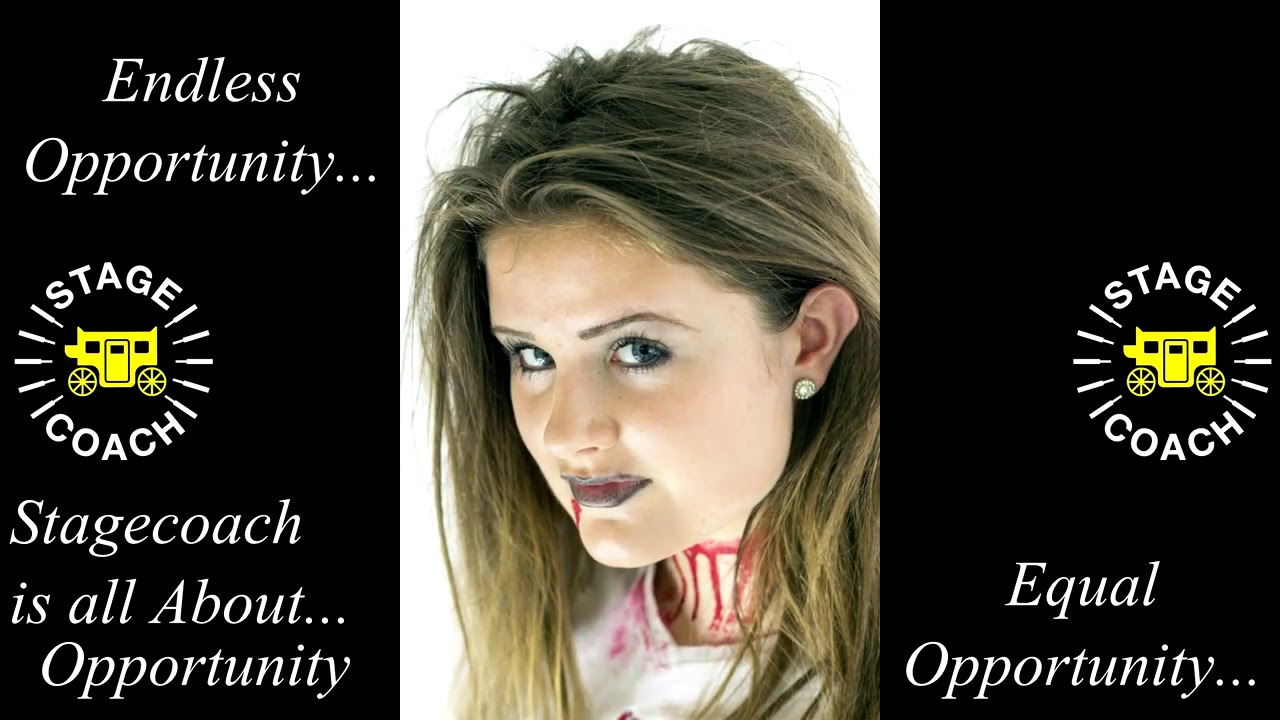This image is an advertisement for "Stagecoach Equal Opportunity," prominently featuring a central picture of a young woman with long, slightly frayed brown hair adorned with earrings. Her striking appearance includes dark makeup, black lipstick, and what seems to be fake blood dripping from her mouth and down her neck, staining her white shirt, giving her a vampire-like or cosplaying look. The background is plain white, making her haunting visage stand out. Flanking her are text and logos: to the left, the words "Endless Opportunity Stagecoach" are accompanied by a yellow, old-fashioned stagecoach symbol, and to the right, a black panel repeats the "Stagecoach" logo and the phrase "Equal Opportunity," reinforcing the theme of opportunity that the advertisement seeks to convey.